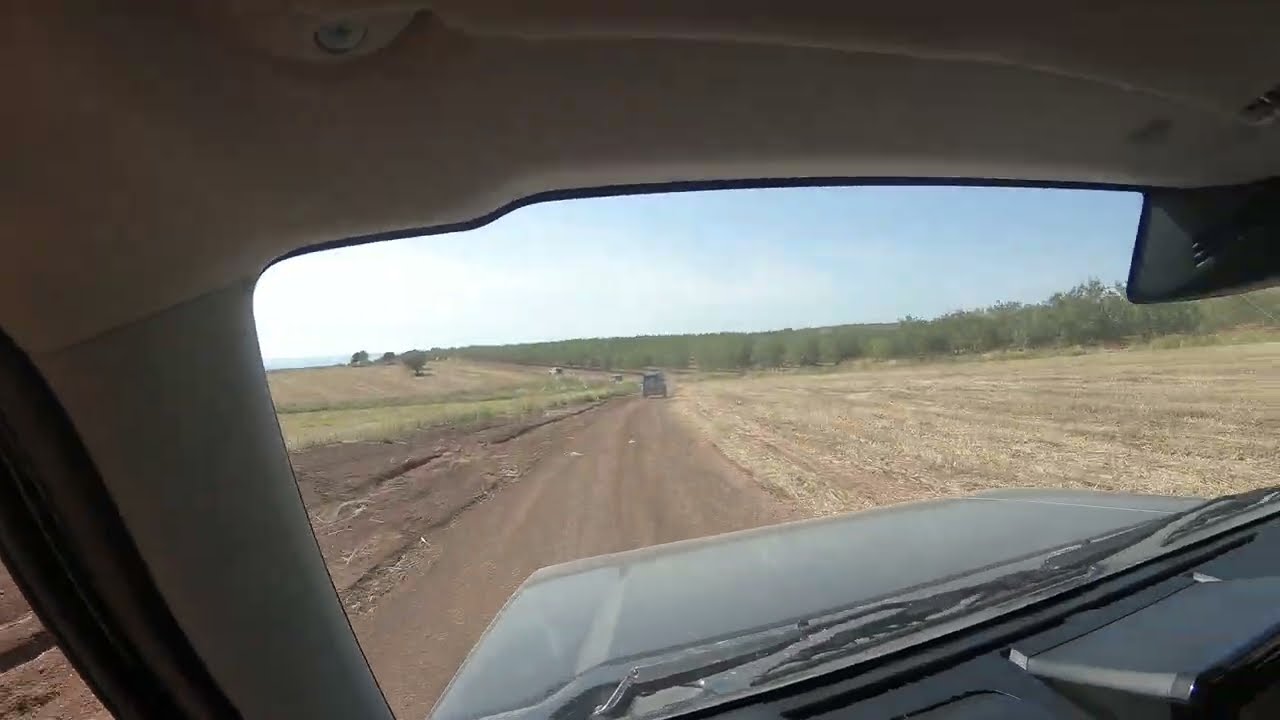This high-definition photograph captures a vivid scene from the driver's seat of a dark-colored vehicle, possibly black or dark gray, with an olive or dark green hood. The image looks out through the windshield onto a narrow, one-lane dirt road. On the left side of the road, a narrow trench runs parallel with dormant yellow and green grass lining it, leading back to a rolling hill where the grass turns even yellower. To the right, the ground is flat, covered with dead yellow and green weeds, possibly remnants of a cultivated field. In the near distance, another vehicle, possibly a van, travels along the road, with two additional cars visible further ahead as the road curves left. In the far distance, a ridgeline of lush, dark green trees with full leaves is visible, under a mostly blue sky that becomes white and hazy toward the left. Inside the vehicle, the view includes the handlebar and the A-pillar on the left, the visor, and a black plastic square hanging near the top of the windshield, with the light brown ceiling above and gray lining on the sides.